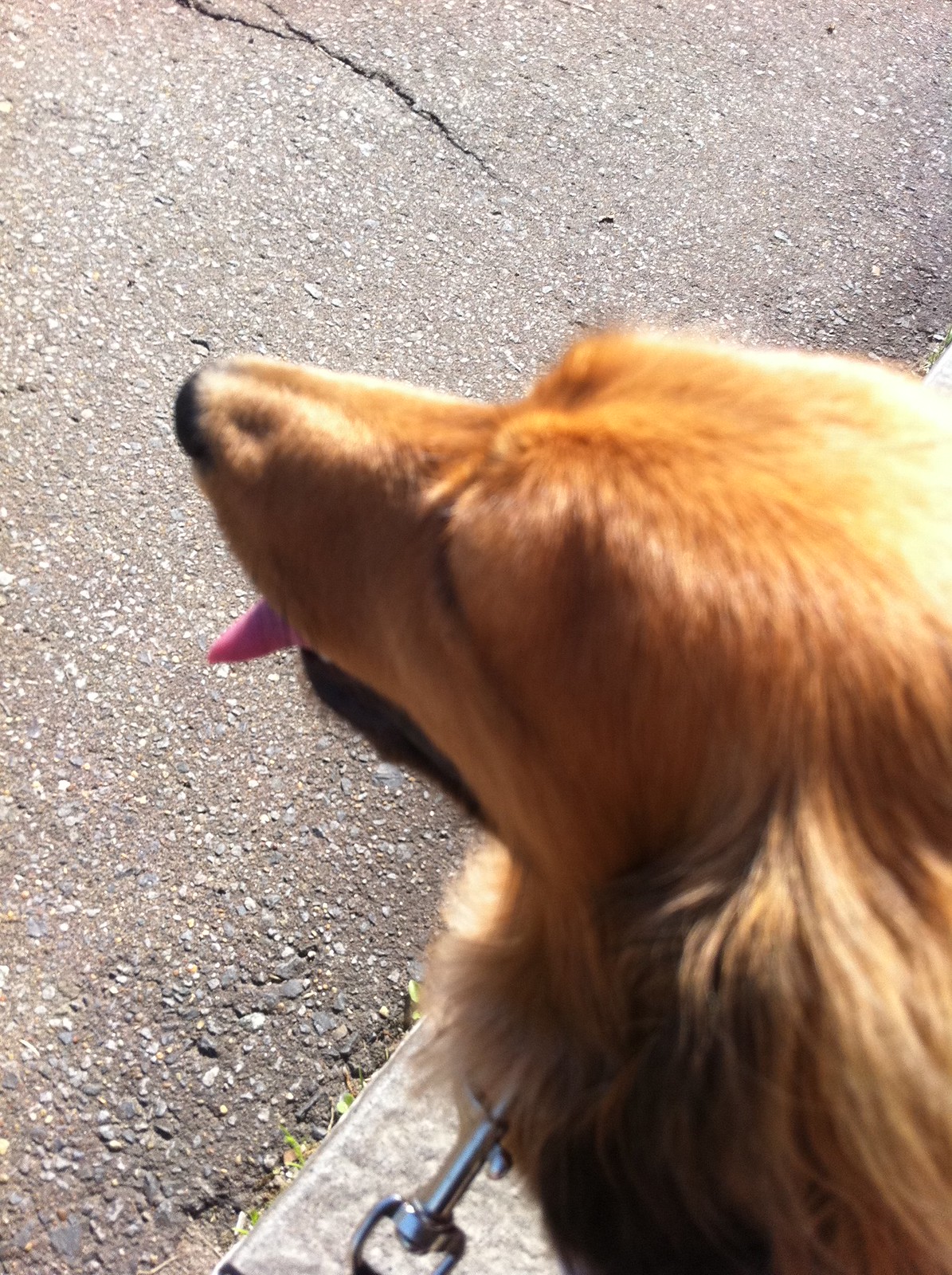The image depicts a caramel brown and gold dog with a skinnier nose, possibly resembling a border collie. The dog’s tongue is pink and hanging out. Despite its thicker fur obscuring a clear view, a leash is evident due to the visible hook, indicating it is attached to a collar underneath the fur. The dog's head, slightly out of focus, is coming in from the right side and facing left. The setting includes a gray cement sidewalk under the dog, transitioning to black asphalt with embedded white and gray pebbles in front of it. This close-up view primarily focuses on the top of the dog’s head and face.